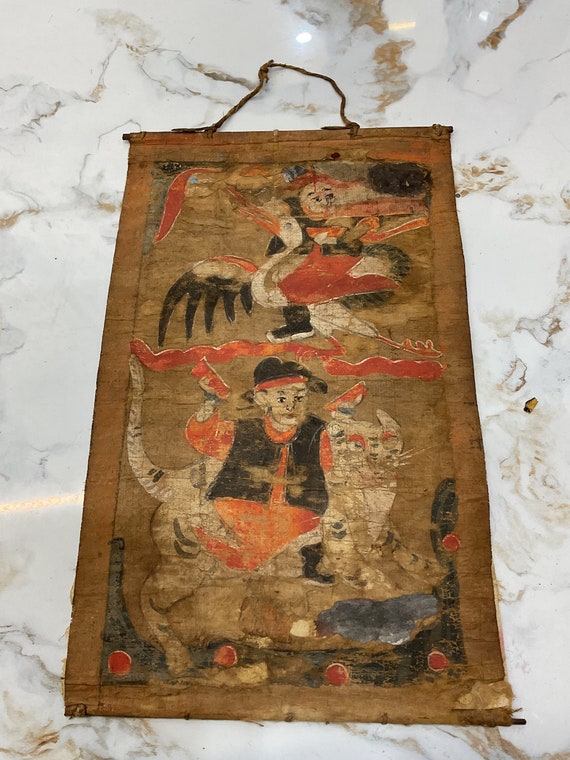The image is of an old, hand-painted scroll or tapestry resting on a white and gold marble countertop. The scroll or tapestry, possibly made of woven fabric or paper mounted on fabric, is tattered and faded due to age. The artwork, likely Asian or Middle Eastern in origin and possibly dating back to the 1800s or earlier, features two main figures painted in white, red, and black. 

The upper part of the scroll depicts a figure, potentially a woman, interacting with a white goose or crane that has black-tipped wings. This person is dressed in black and red clothing. The lower part of the scroll shows a man standing next to a white tiger with black stripes. He's dressed in a black vest over an orange shirt, red pants, black boots with white soles, and a black hat with a red band. He holds red objects in each hand, and there appears to be an element resembling fire separating the two figures. The artwork's details are marred by its worn and dirty state, which makes some elements difficult to discern.